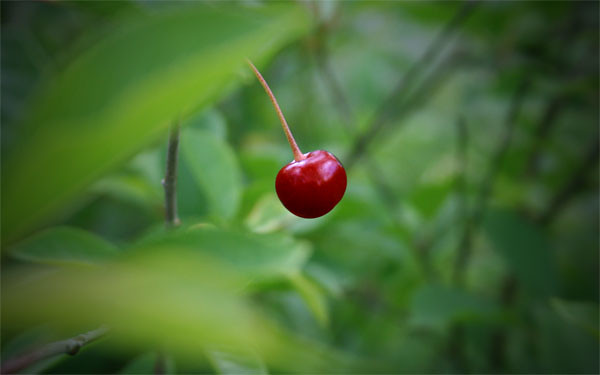This is a full-color, staged photograph taken outdoors on a sunny day, capturing the vibrant essence of nature. In a lush, green forest teeming with blurred foliage, the focus is a single cherry hanging from a tree. The cherry, possibly of a unique variety due to its slightly asymmetrical shape, boasts a striking combination of bright red and burgundy hues, glistening under the sunlight. Its long white stem adds an additional focal point as it dangles from a green branch. The environment is rich and moist, evidenced by the vibrant green leaves and long, thick brown stems of the surrounding foliage. Despite the complexity of the background, the solitary cherry commands attention as the central subject of the photograph, accentuated by the contrasting greenery that frames it.